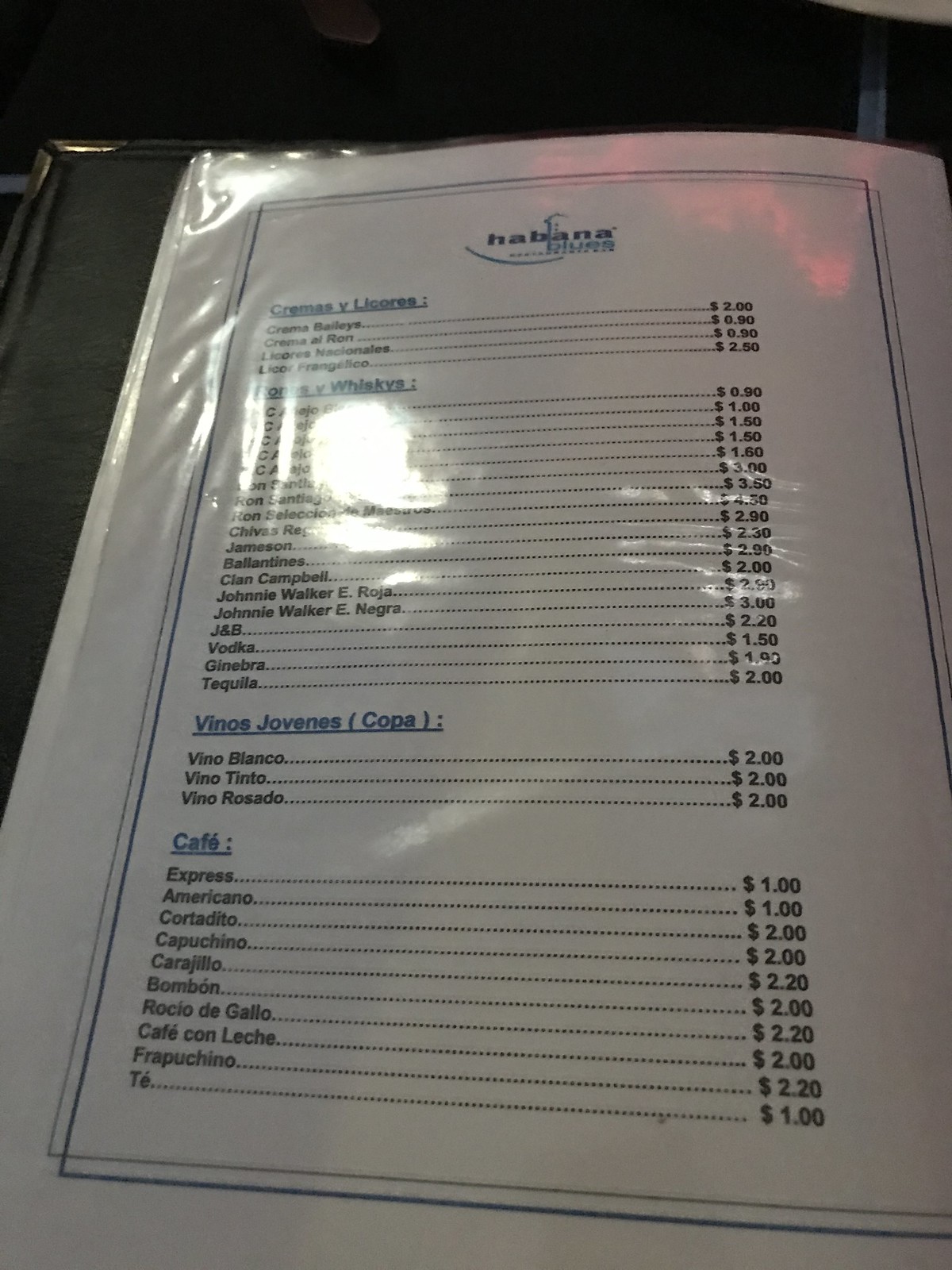This image showcases a single page from a larger menu booklet. The menu is printed on a long, white, legal-sized paper, and it is inserted into a protective plastic sleeve, which is part of the menu's overall binding. The menu features a blue and black color scheme with blue titles for different sections and black text detailing the items and their prices. 

In the top center, the word "Habana" is prominently displayed in bold letters, with some illegible blue text underneath it. There is also a small illustration, possibly of a house. Below this heading, additional text in Spanish appears, indicating various categories or offerings, potentially reading "versus licores". 

In the left corner of the image, the black and gold outline of the menu's cover is partially visible, indicating the edge of the full menu booklet. A glare, likely from a nearby window, disrupts the view of the menu's contents, making them difficult to read. The overall image is fuzzy and out of focus, further obscuring the detail.